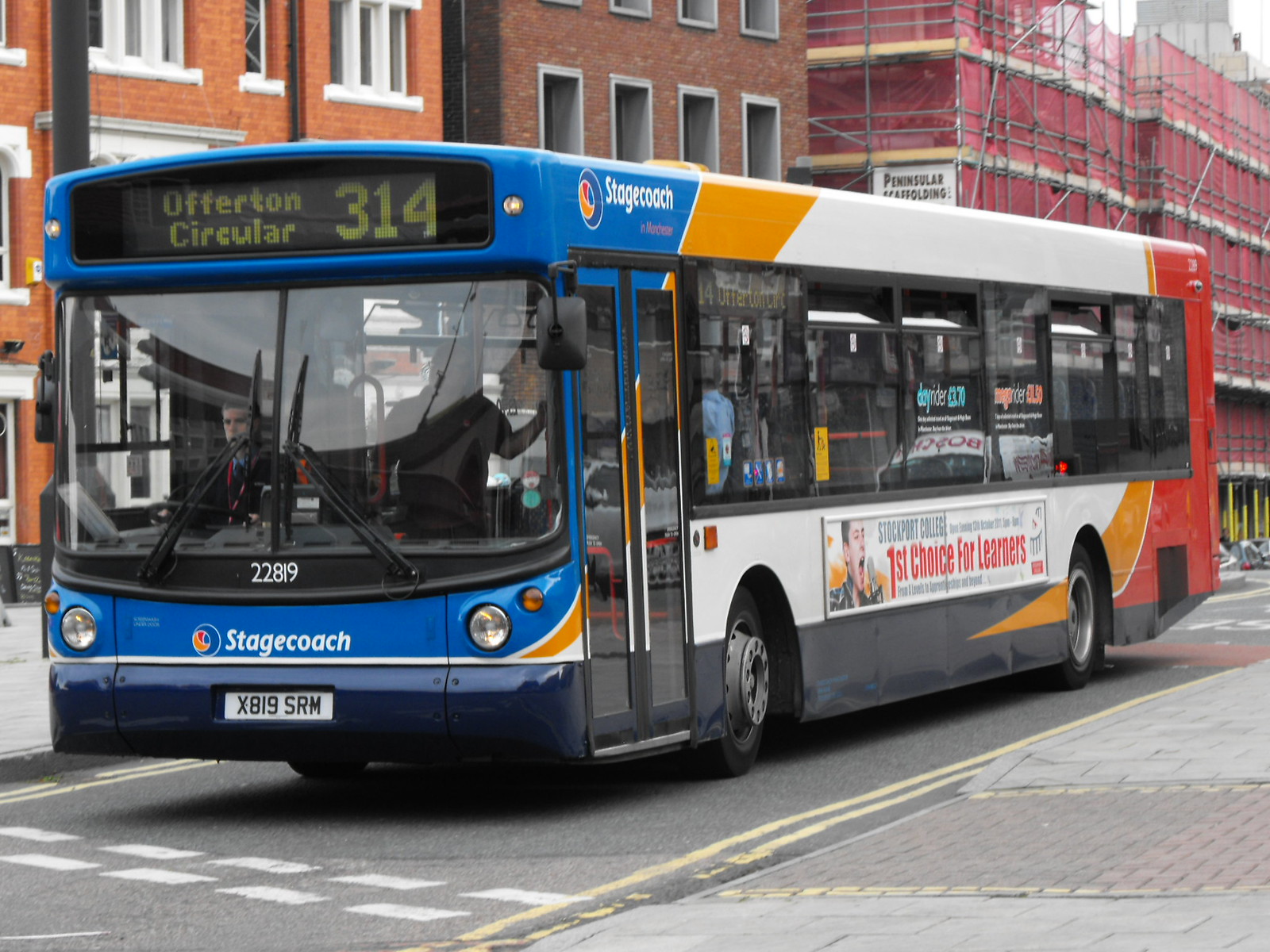The image captures a bustling city street scene in England. Dominating the foreground is a blue city bus identified as part of the Stagecoach fleet, with the license plate X819SRM and the bus number 22819 prominently displayed. The bus's digital sign at the top reads "Offerton Circular 314" in green letters. A bus driver sits on the right-hand side, fitting the standard UK setup. At the exit door, a gentleman stands poised to disembark. The bus's exterior features an ad with the slogan "First choice for learners." The roadway is marked with white striped lines and yellow road lines. Surrounding the scene, a red brick building creates a vivid backdrop, stretching from left to right, with variations in the brick color from orange to a darker shade. Sidewalks flank the street on both sides. In the further background, there's a hint of a storage or construction area. The scene is captured during the daytime, with the clean and busy street reflecting city life.